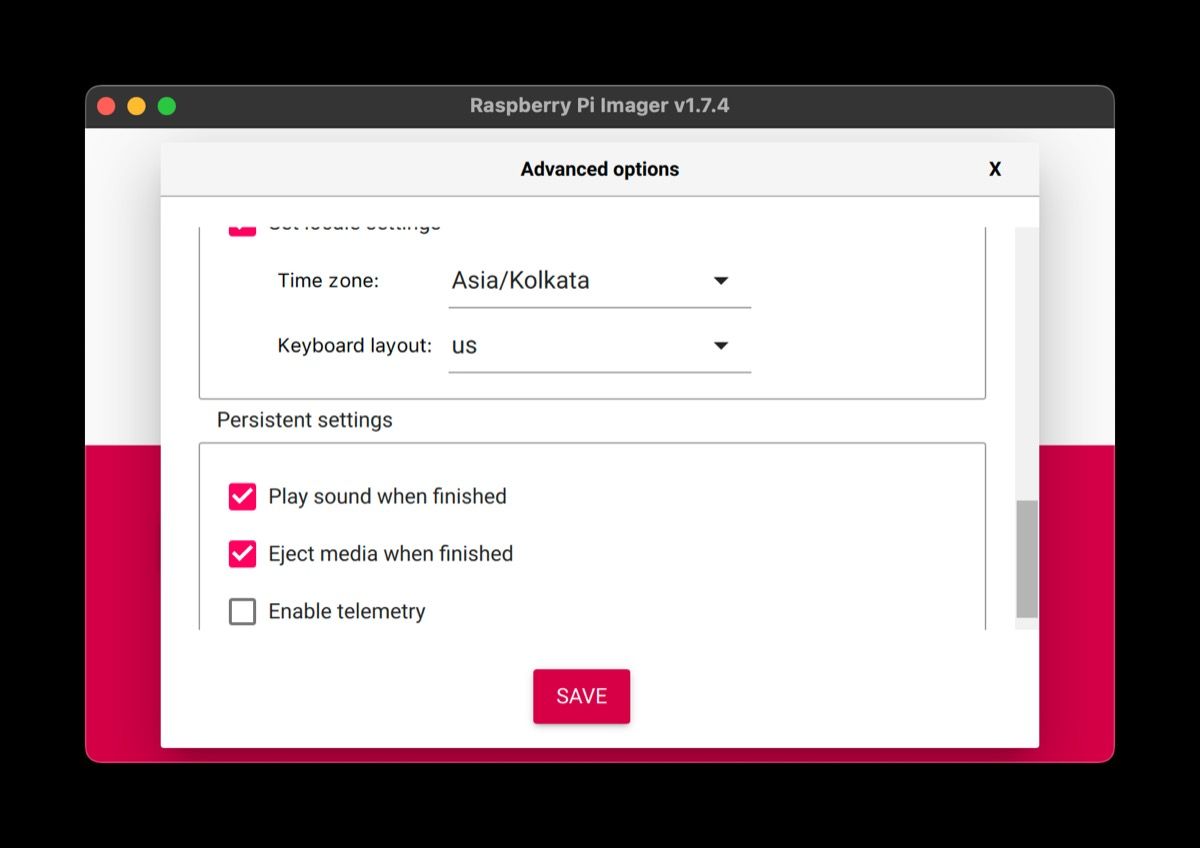Here is a cleaned-up and detailed caption for the image:

---
The image is a screenshot of a window displaying the "Raspberry Pi Imager V1.7.4" software interface. The background is a solid black, with the software window prominently in the foreground. The software window has a black header with red, orange, and green buttons on the left side, resembling traditional window control buttons. Below the header, the window is divided into two main sections.

The top part of the window is white and features a tab labeled "Advanced Options." Within this section, specific settings are detailed. The time zone is set to "Asia/Kolkata," and the keyboard layout is specified as "US."

Beneath the white section, the interface has a raspberry-colored background. This lower section is titled "Persistent Settings" and includes several checkbox options:
- "Play sound when finished," which is checked and denoted by a white check mark in a raspberry-colored box.
- "Eject media when finished," also checked with a similar raspberry-colored box and white check mark.
- "Enable Telemetry," which remains unchecked.

At the very bottom of the window, there is a prominent raspberry-colored button with white text that says "Save."

The overall design is clean and functional, with clear sections and options to enhance user interaction with the Raspberry Pi Imager software.
---

This caption provides a detailed and organized description that is easy to understand.